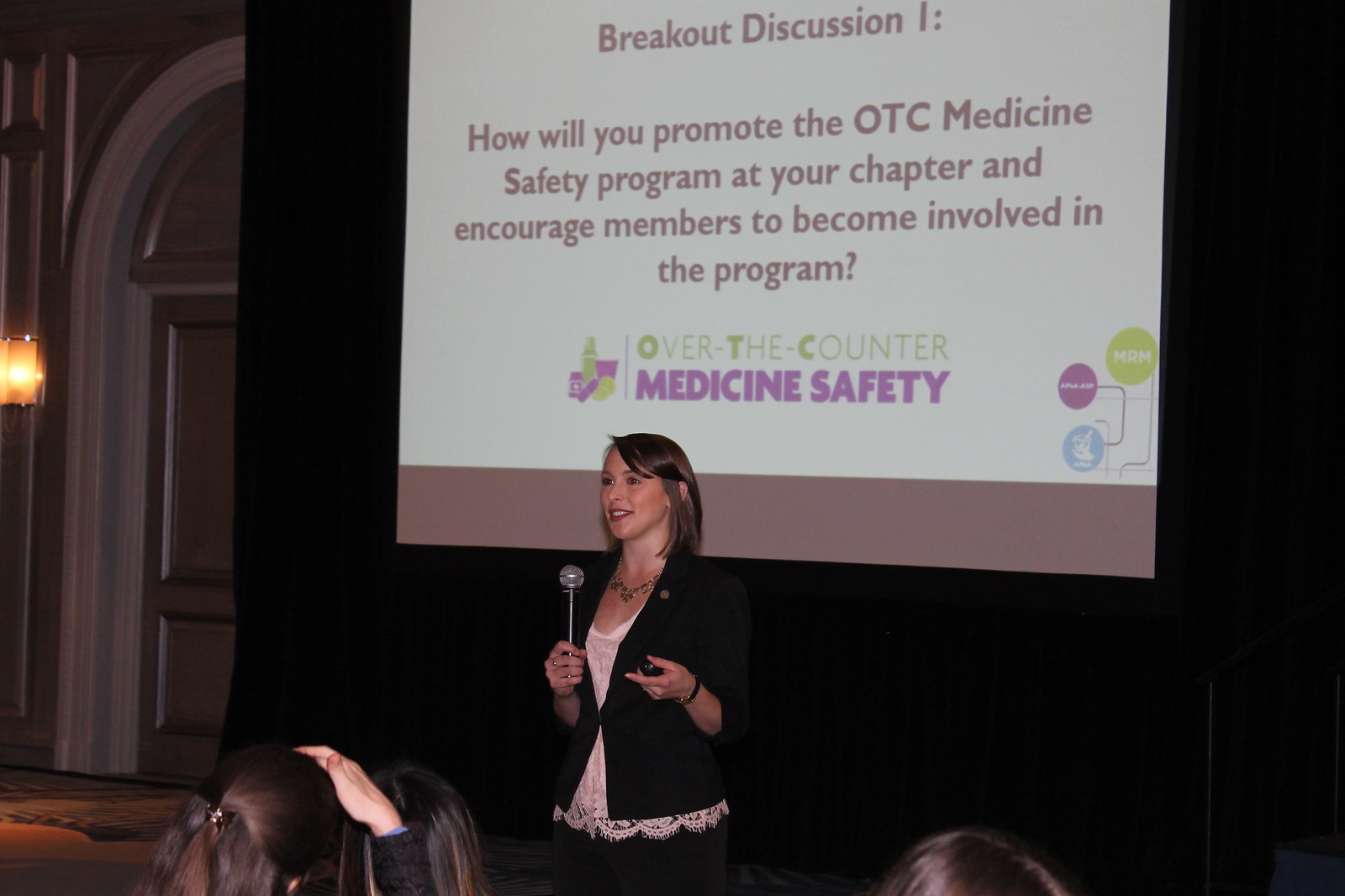In this vibrant color photograph, a smiling woman stands at the center, engaging with the crowd in front of her. Her hair is parted on the left, flowing over her right ear, which is partly visible. She is dressed in a black jacket over a white shirt and accessorized with a necklace. Holding a black microphone in one hand, the woman addresses the audience with her other hand raised to stomach level. The microphone gleams with a sliver of light, catching the ambient illumination.

Behind her, a white banner adorned with vibrant designs and text dominates the background. The banner prominently features the title "Breakout Season 1: How Will You Promote the OTC Medicine Safety Program at Your Chapter and Encourage Members to Become Involved in the Program?" in purple text. Beneath this, "Over-the-Counter Medicine Safety" is written in alternating green and purple letters. The right side of the banner is embellished with three interconnected circles containing words, adding a dynamic visual element.

In the audience, the backs of several heads are visible, including a distinct figure with a hand resting atop their head. The scene is further framed by an orange light glowing from the far left and an arched doorway with a lamp mounted on the wall. This meticulously composed scene captures a moment of active engagement and purposeful dialogue.